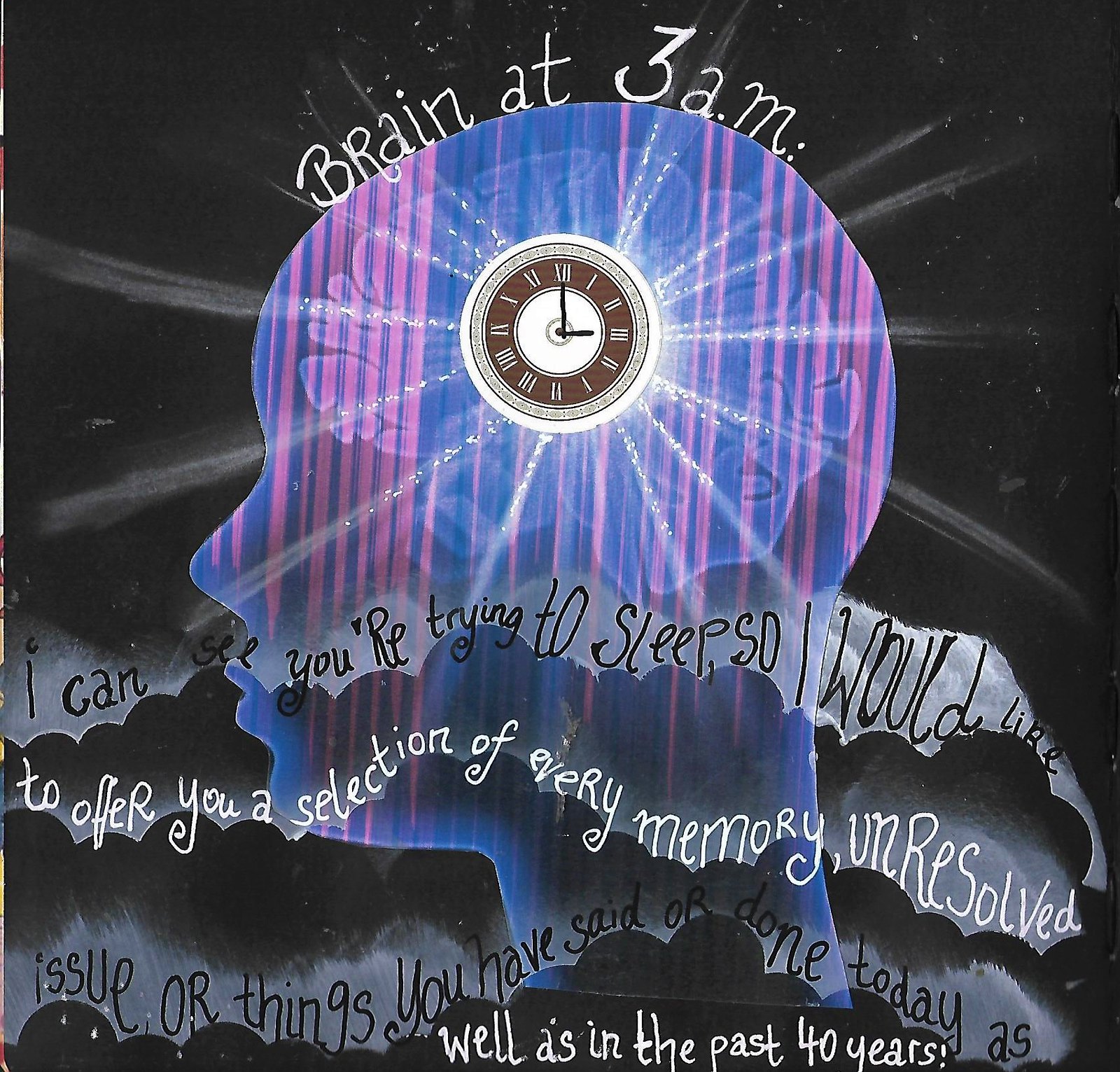The image is a square piece of abstract digital artwork with a black background adorned with tiny white dots resembling stars. The main subject is the side profile of a bald human head, which is transparent and colored in various shades of blue and purple with vertical pink stripes. In the center of the head, where the brain would be, there is a large clock with Roman numerals set at 3 o'clock, and emanating light rays.

At the top of the head, in bold white letters, it reads: "Brain at 3 a.m." Below the clock, there is a lengthy text written in alternating black and white letters that humorously states: "I can see you're trying to sleep, so I would like to offer you a selection of every memory, unresolved issue, or things you have said or done today, as well as in the past 40 years!"

The bottom of the image features several white outlines of clouds near the mouth and neck area of the head, adding to the surreal and dream-like quality of the piece. The text appears handwritten, contributing to the personalized and whimsical nature of the artwork, which vividly captures the chaotic and restless state of a brain at 3 a.m.